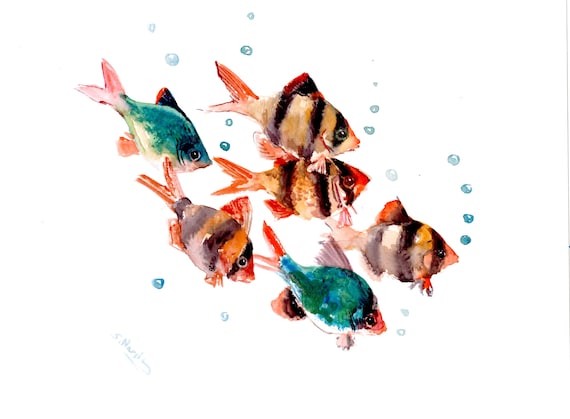A vibrant watercolor painting on a white background showcases six tropical fish, swimming diagonally from the top left to the bottom right. The grouping includes two teal fish with orange tails and four tiger-striped fish in shades of white, black, and orange. Each fish has distinct bubbles, varying in shades of blue, emerging from their mouths, giving the illusion of movement through water. The fish exhibit large, expressive black eyes and small fins. The striped ones have prominent black stripes running vertically across their bodies, and all sport bright orange or reddish tails. The artist's subtle, yet finely detailed, semi-realistic style captures the colorful essence of the fish. The painting is signed in a light blue color in the bottom left corner.